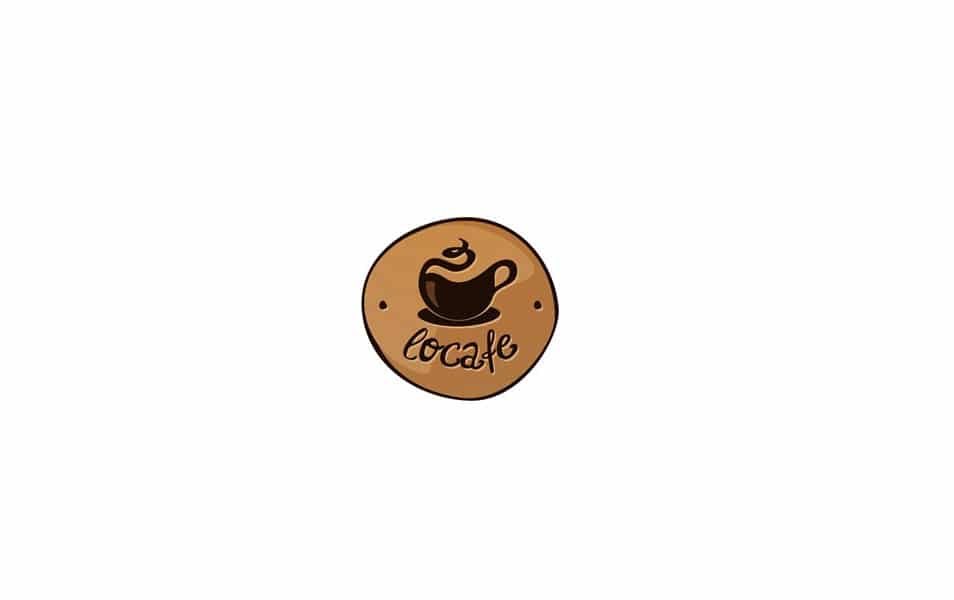The image features a coffee shop emblem centered on an all-white background. The emblem itself is a small, slightly imperfect circle with a dark brown wobbly border. Inside this circle, the background is a lighter brown or tan color. At the center, there is an artistic drawing of a coffee cup with a handle on the right. The cup is distinctive for its curlicue design on the left side, suggestive of swirling steam. Flanking the coffee cup are two dark brown dots, one on the left and one on the right. Beneath the coffee cup, in cursive dark brown letters, is the text "LOCAFE." The cup and text also exhibit a shading effect, appearing lighter at the top and darker at the bottom, giving a sense of depth and reflection. Overall, the emblem employs a simple yet reflective artistic style, making it the focal point of the minimalist design.